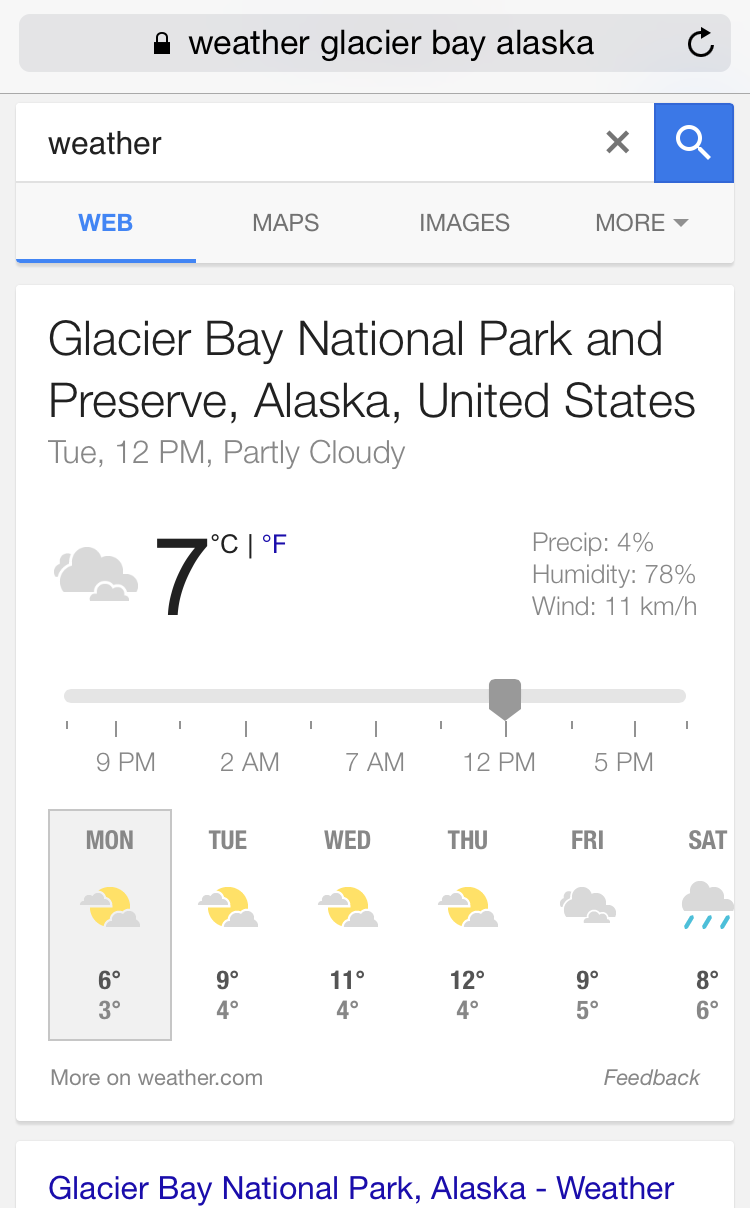The image depicts a weather forecast interface for Glacier Bay National Park and Preserve, Alaska. At the top, there's an address bar featuring a lock icon and the label "Weather, Glacier Bay, Alaska," indicating a secure connection. Below the address bar is a search box with a placeholder text reading "weather." Following that, there are tabs labeled "web," "maps," "images," and "more."

A prominent white box displays key weather details: 

- Location: Glacier Bay National Park and Preserve, Alaska, United States
- Time: Tuesday, 12pm
- Condition: Partly cloudy
- Temperature: 7 degrees (both Celsius and Fahrenheit), with Fahrenheit highlighted in blue

Additional weather metrics include:
- Precipitation: 4%
- Humidity: 78%
- Wind: 11 km/h

Below these details, there's a sliding bar chart spanning from 9pm to 5pm the next day, currently positioned at 12pm. This is followed by a seven-day weather forecast:

- Monday: High 6°C, Low 3°C
- Tuesday: High 9°C, Low 4°C
- Wednesday: High 11°C, Low 4°C
- Thursday: High 12°C, Low 4°C
- Friday: High 9°C, Low 5°C
- Saturday: High 8°C, Low 6°C